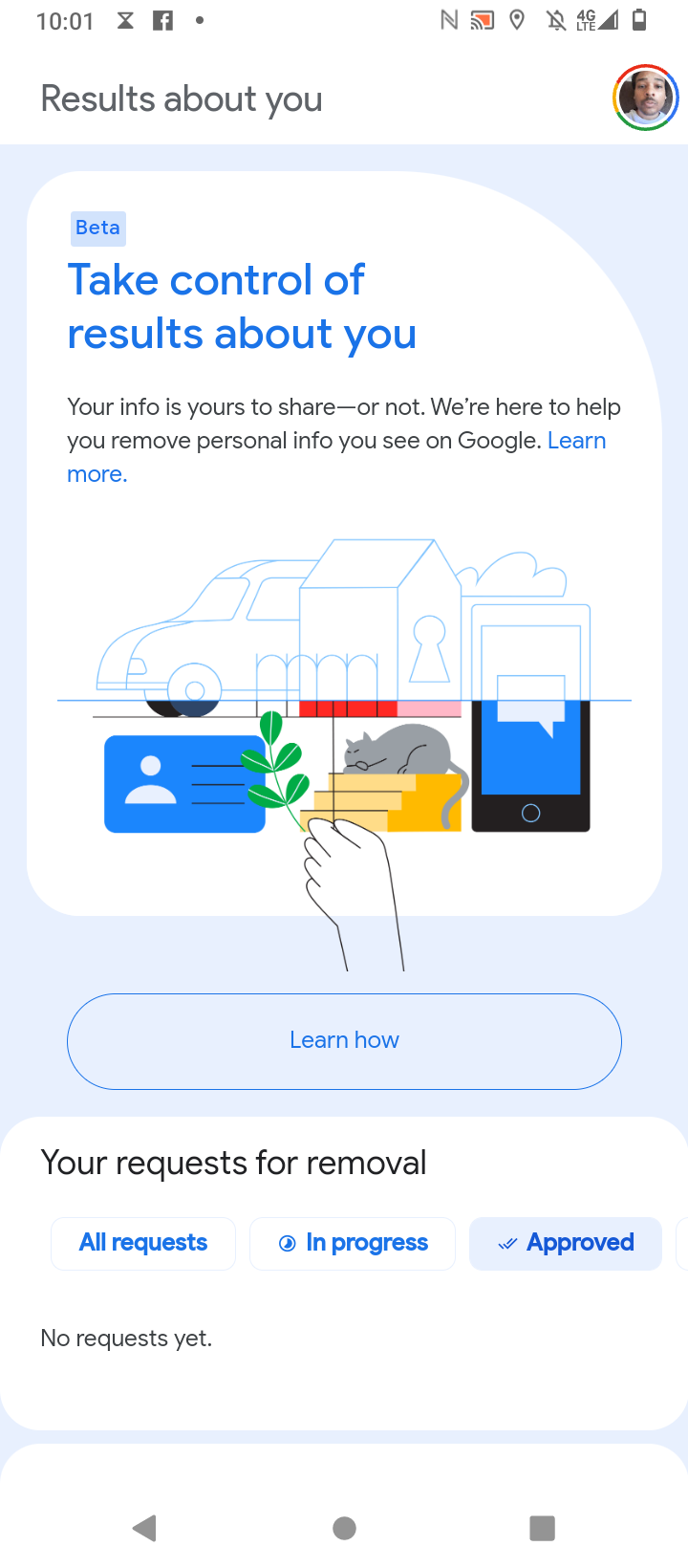The image appears to be a screenshot taken from a smartphone, featuring a mobile interface. The screenshot includes multiple elements neatly organized within the mobile screen’s typical layout.

At the top of the image, there's a white toolbar displaying various icons and information. On the left side, the number '1001' is presented in small black text, adjacent to an hourglass icon filled with black at the bottom. Following that is the familiar Facebook 'F' icon. On the far right of the toolbar, several icons appear aligned: an 'N' icon, a square-shaped Wi-Fi signal icon on an orange background, a GPS marker, a muted bell symbol indicating notifications are silenced, the '4G LTE' label indicating network connection, another internet connectivity bar symbol, and a battery icon showing half charge.

Below this toolbar, the title "Results about you" is prominently placed on the left upper side, contrasted on the right by a circular avatar of a black man.

The main portion of the screenshot is dominated by a light blue rectangular section. Inside it sits a white speech bubble containing the text "beta" in blue, followed by "Take control of results about you" in black letters. Below this text, it states, "Your info is yours to share or not. We're here to help you remove personal info you see on Google." A "Learn more" link appears in blue.

Moving further down, there are illustrations: an outlined drawing of a car and a house with a keyhole, featuring a garage. Following this illustration is a colored image of a black ID card with a white stickman figure marking a person's head and shoulders. Adjacent to this image are three brown steps with a gray cat sleeping atop them. On the right side, part of a smartphone is visible, though partially cut off. A hand-drawn figure holding a twig of green grass is positioned in front of the steps.

Towards the bottom, a large blue oval button labeled "Learn How" is visible, followed by another white rectangular section that reads, "Your request for removal" in black font. Several blue buttons appear below this text: "All Requests," "In Progress," and "Approved," with the latter highlighted in a darker blue hue and marked with a check mark. Beneath these buttons, the words "No Requests Yet" are visible.

Finally, at the very bottom of the screenshot, there are playback control icons: a play button facing left, a circular record button, and a square stop button.